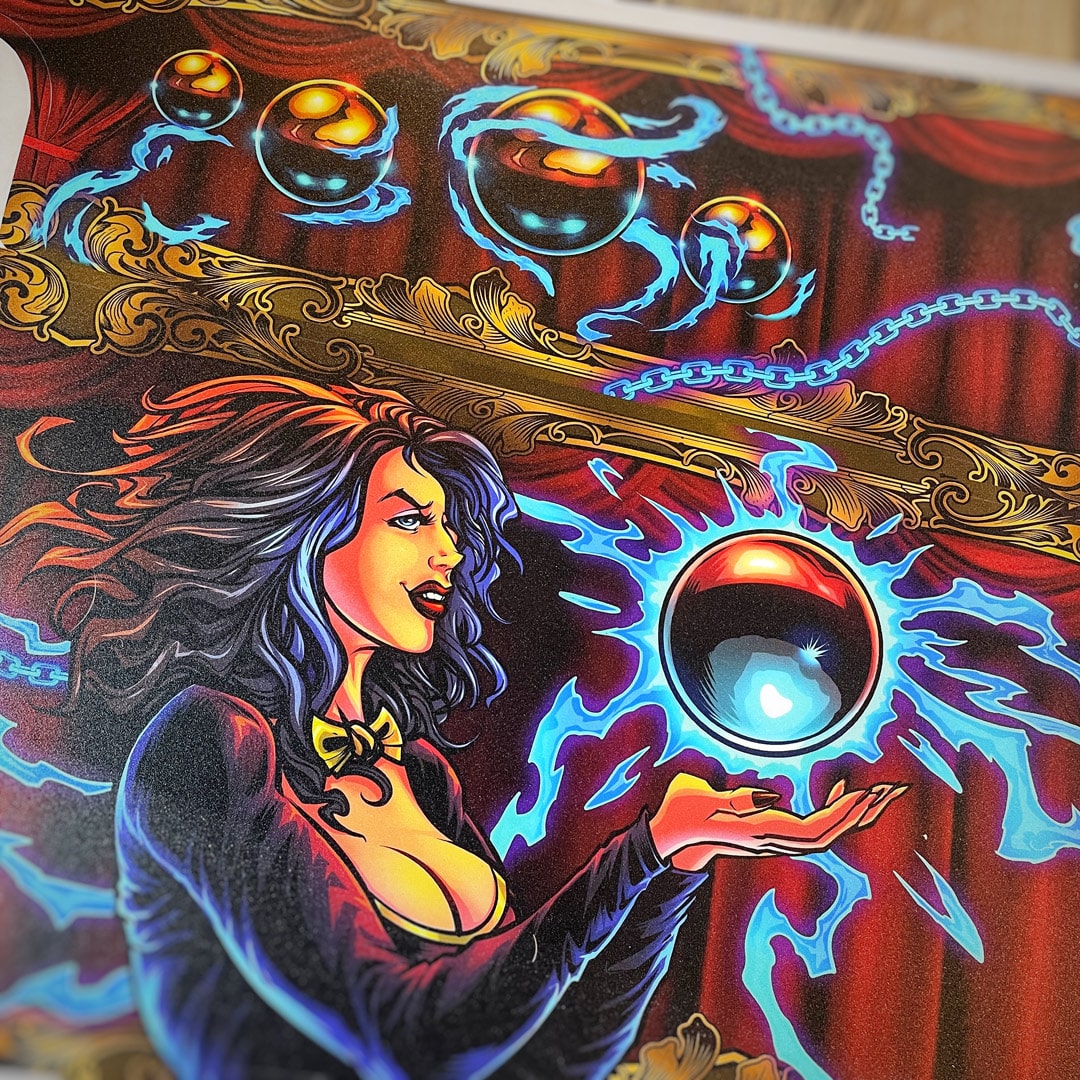The image is an illustration with a cartoon style, featuring a woman with a pretty face and an evil grin, possibly a witch or a fortune teller, with disheveled blackish-blue hair whipping backwards. She has red lipstick and is wearing a low-cut black dress with a yellow bowtie. The woman is demonstrating her magical powers on a stage, indicated by the red theater curtains with a gold stripe in the background, suggesting it is an indoor setting. She is holding a large, levitating crystal ball just above her palm, which radiates blue electrical energy and fire from within. Above her, four additional metallic crystal balls, also emitting blue lights and fiery effects, hover in the air, showcasing her telekinetic abilities. The scene suggests she is performing a mystical act, captivating the audience with her supernatural spectacle.